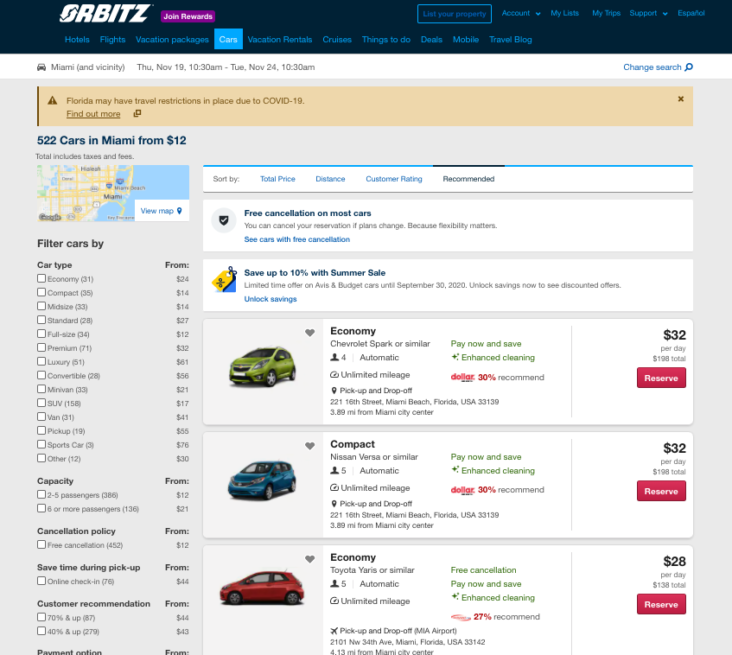Screenshot of the Orbitz Car Rental Site: 

The image captures the Orbitz car rental site. At the top, a black banner prominently displays the Orbitz logo, accompanied by a purple "Join Rewards" button. The navigation menu highlights various categories: Hotels, Flights, Vacation Packages, Cars (selected), Vacation Rentals, Cruises, Things to Do, Deals, Mobile, and Travel Blog. 

Beneath the navigation menu, an orange alert banner warns, "Florida may have travel restrictions in place due to COVID-19, find out more." Below the alert, it states, "522 cars in Miami from $12." 

The interface continues with a small map screenshot and filtering options for cars. Users can filter based on car types, capacity, cancellation policy, save time during pickup, and customer recommendations. To the right of the map, there are sorting options: total price, distance, customer rating, and recommended.

Additionally, a banner offers "Free cancellation on most cars" and promotes savings of up to 10% with the summer sale. The interface displays three images of small sedan-type cars: a green car labeled as "Economy" for $32, a blue car also labeled as "Compact" for $32, and a red car labeled as "Economy" for $28. Each listing includes further details in small text below the car images.